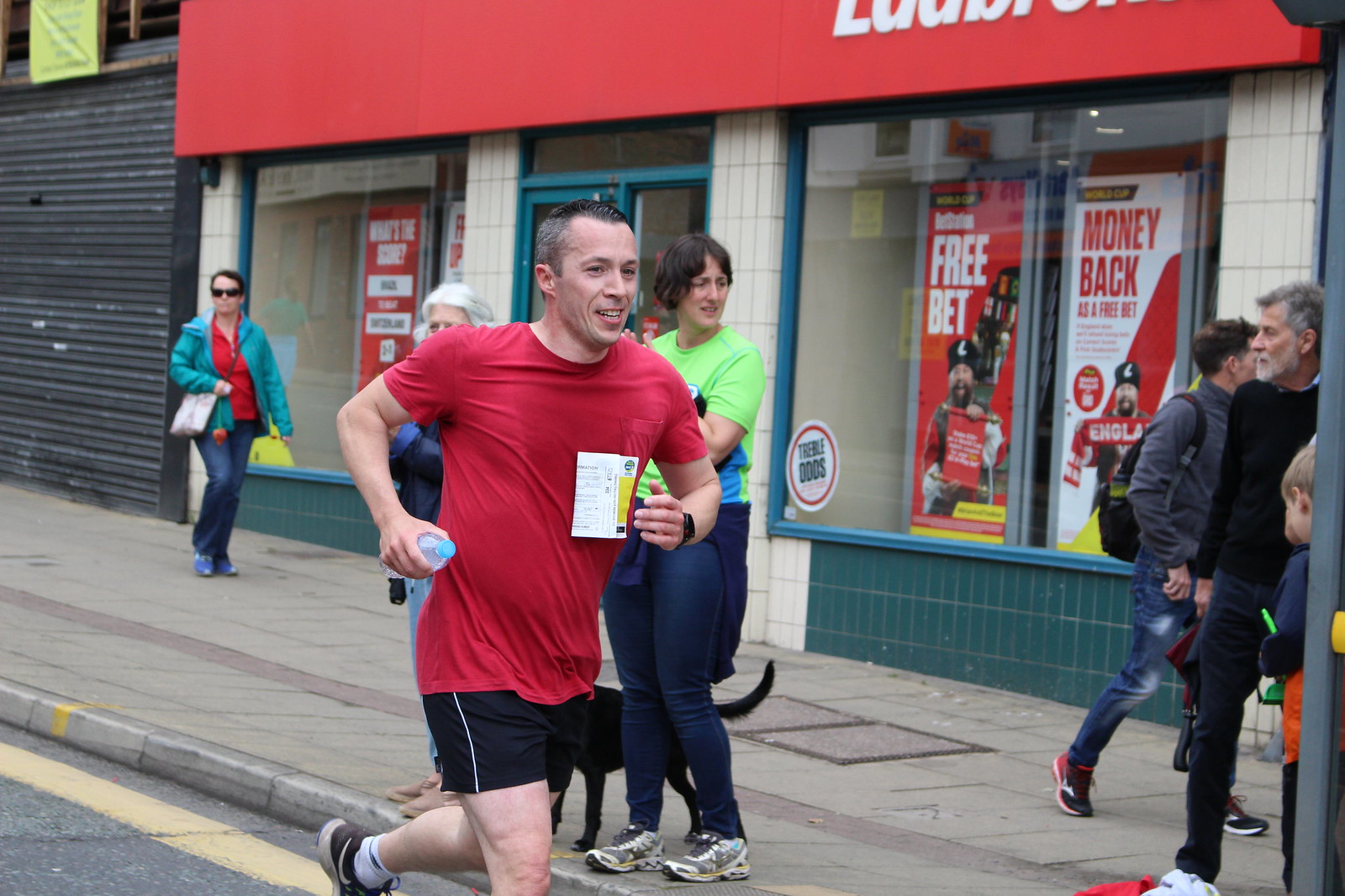This rectangular outdoor photograph captures the spirited action of a marathon or running race. Dominating the center of the image is a middle-aged man, likely in his 40s, with short salt-and-pepper hair. He is actively mid-run, smiling, and appears to be enjoying the event. Clad in a sweat-soaked red t-shirt with what seems to be his registration number affixed, he holds a water bottle in one hand, his arms swung naturally beside him. He is wearing black shorts, black running shoes, and white socks, running on an asphalt road marked by the yellow paint of the boundary lines.

In the background, the scene is framed by a sidewalk lined with stone tiles. Several spectators and pedestrians populate this area, adding to the lively atmosphere. Among them, notable characters include a woman in a green shirt and leggings standing with a black dog, and another woman in a green coat and red shirt holding a shoulder bag. A bearded man with gray hair, dressed in a black sweater and dark pants, is also visible. Behind them, a series of storefronts display various advertisements, including prominent red and white signs reading "Free Bet" and "Money Back." The array of colors—gray, yellow, red, black, tan, light green, dark green, and blue—adds vibrancy to the scene, confirming it is a sunny day in an urban environment.